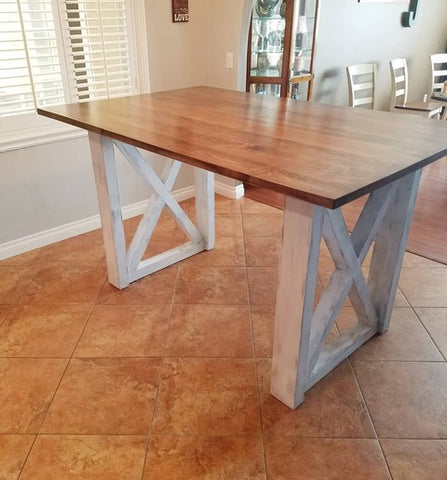The image showcases the interior of a warmly lit dining room, dominated by a substantial table placed at its center. The table features a thick, medium brown, glossy wooden surface that shines with a polished finish. The sturdy legs of the table are composed of weathered, white-painted wood arranged in an intricate design with rectangular forms and X-shaped cross beams, giving them a rustic, reclaimed wood appearance. The flooring beneath the table consists of orange-brown tiles, contrasting with the table's refined texture. In the top right corner of the image, there are three chairs positioned in front of a butler cabinet shelf. This adjacent room, distinguishable by its brown wooden flooring, also features walls painted in a calming gray tone, and horizontal white blinds shade a window in the top left corner of the image. A glass display case to the left, filled with glasses and vases, also captures attention, adding to the room's sophisticated decor.